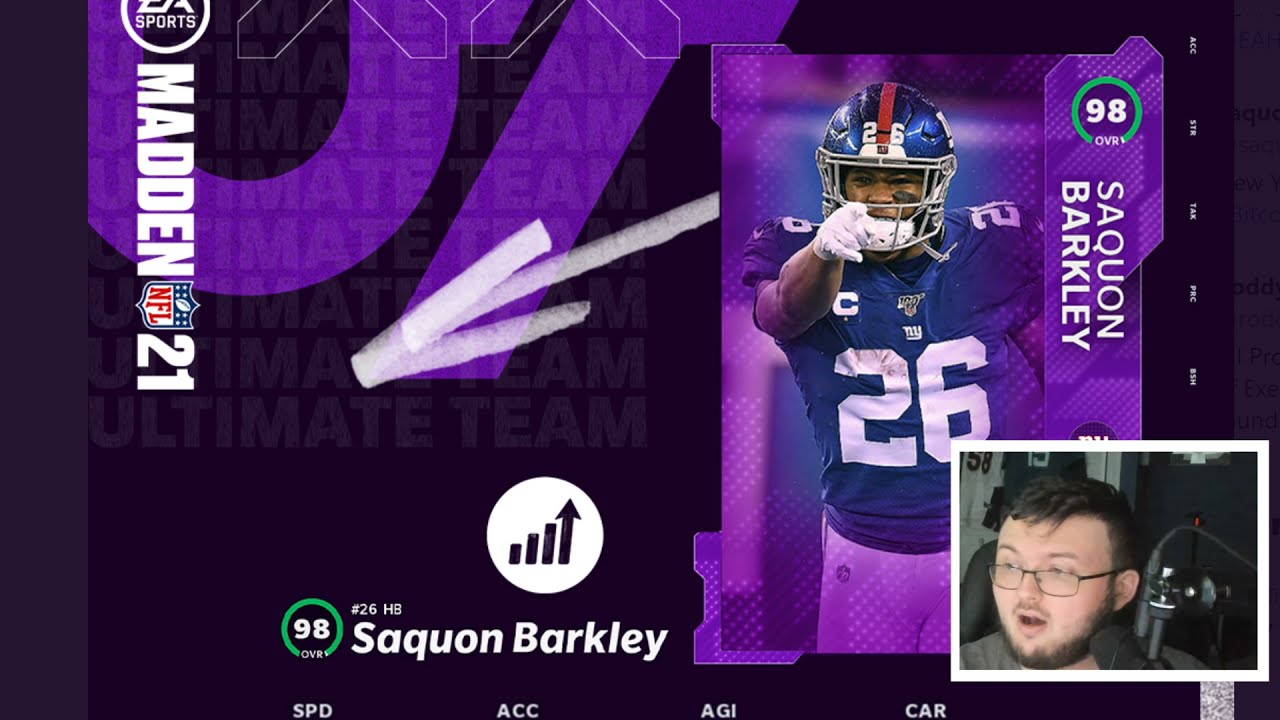The image is a detailed promotional poster for the video game Madden NFL 21, prominently featuring the football player Saquon Barkley from the New York Giants. Saquon is depicted in the center wearing his full uniform: a blue helmet, blue jersey with the number 26, and white pants. He is pointing directly towards the viewer with his left hand, set against a rectangular purple background with a white arrow pointing to the left. To the right of his image, his name, "Saquon Barkley," is clearly displayed along with the number 98, indicating his in-game rating. The text "Madden NFL 21" runs vertically along the left side. In the bottom right corner of the image, there is an inset picture of a person, who appears to be a gamer or podcaster. This individual, who is wearing glasses and talking into a microphone, is sitting in a room, possibly streaming or recording content related to the game. His facial expression suggests he is engaged and possibly commenting on Saquon Barkley's stats or performance. The overall design of the poster, including the white-bordered inset and various textual elements, emphasizes both the featured athlete and the game's branding.